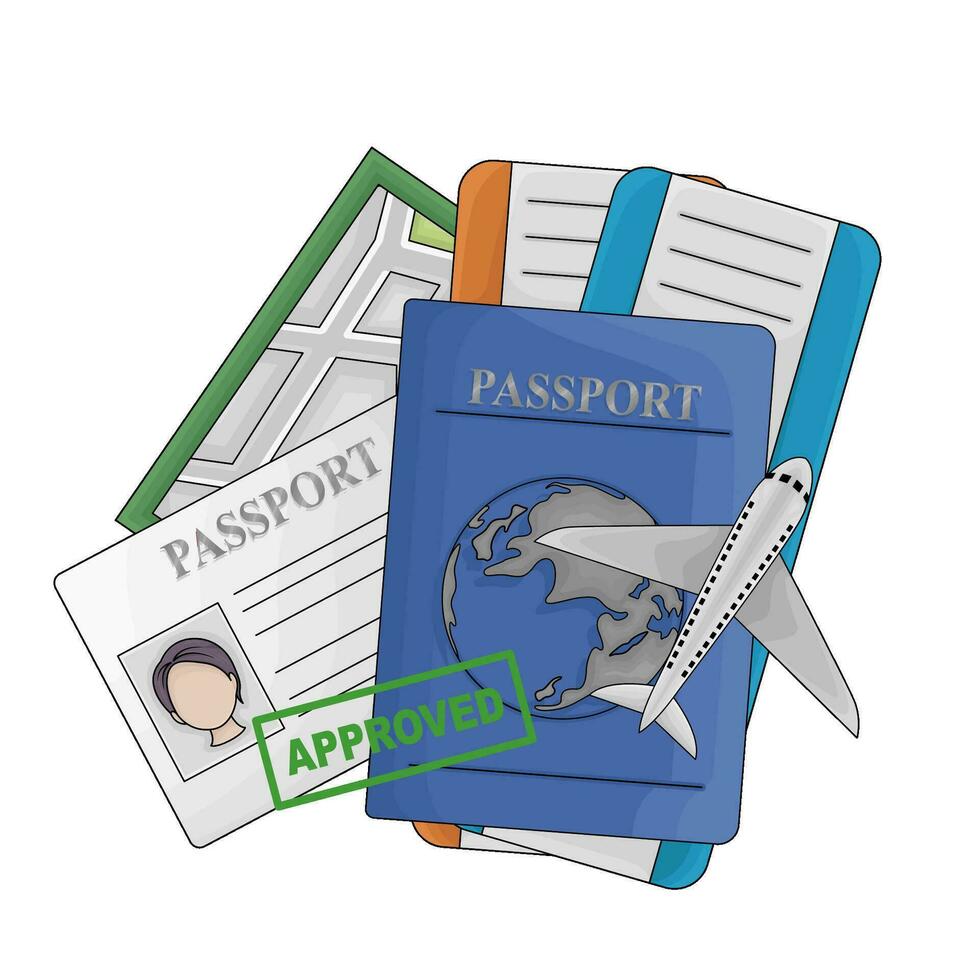This image is a detailed, hand-drawn illustration focused on travel preparation. At its base lies a map with a green border and intricate, gray roadways. Layered atop the map are several travel-related items, including a closed, blue passport book featuring a silver globe emblem and the word "PASSPORT" in capital letters. Next to it is an identification card-like open passport with the word "PASSPORT" in gray at the top, a blank face sketch of an individual with brown hair on the left, and text lines on the right.

Further above, there are two airline tickets; the lower one has an orange trim, while the top ticket is bordered in blue, both featuring white centers with black text lines. A cartoony, toy airplane with visible windows is placed atop these items. Dominating the composition is a slightly crooked, green rectangular stamp with the word "APPROVED" in capital letters, signifying readiness for travel. The overall aesthetic is playful and cartoon-like, encapsulating the excitement and anticipation of embarking on a journey.